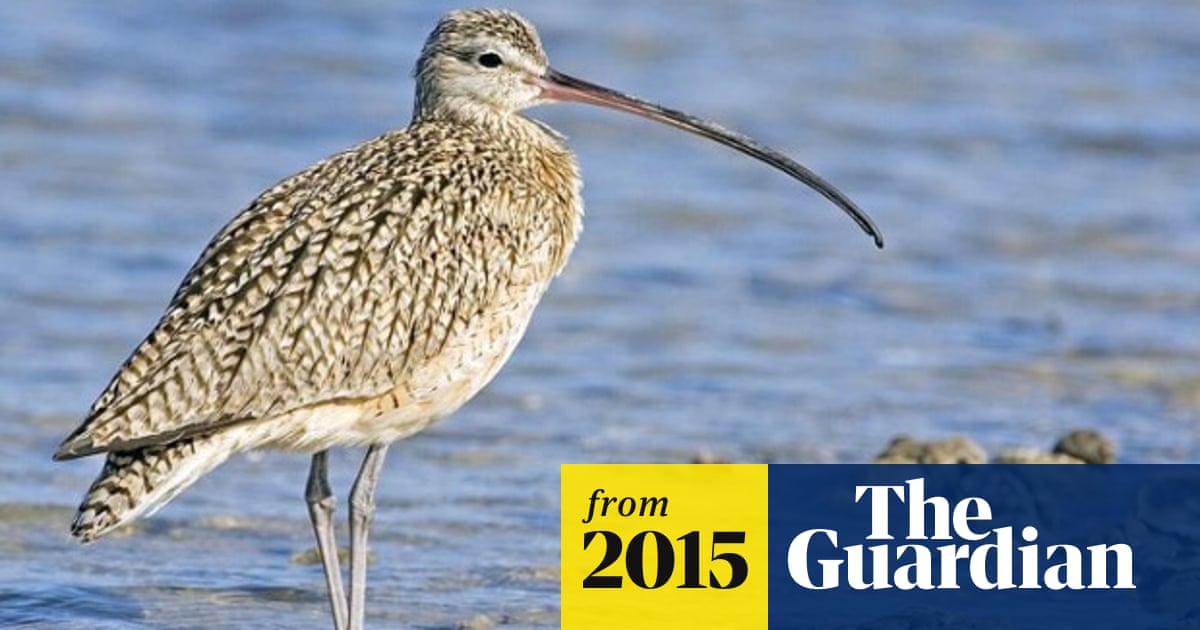The daytime photo features a pelican standing in shallow water, occupying the entire left side of the image. The bird, characterized by its long, thin, and somewhat curved beak that transitions from black at the tip to red closer to its head, has a small head with black eyes and thin gray legs. Its plumage comprises a mix of white with dark lines, brown, and black splotches, especially on its back. The water in the foreground is filled with rocks and has ripples that appear a bit blurry. The background is blurred, bringing the pelican into sharp focus. In the bottom right corner, there's a blue and yellow square logo, where the yellow box contains black text stating "from 2015," and the blue box features the white text "The Guardian," indicating the photo's source.